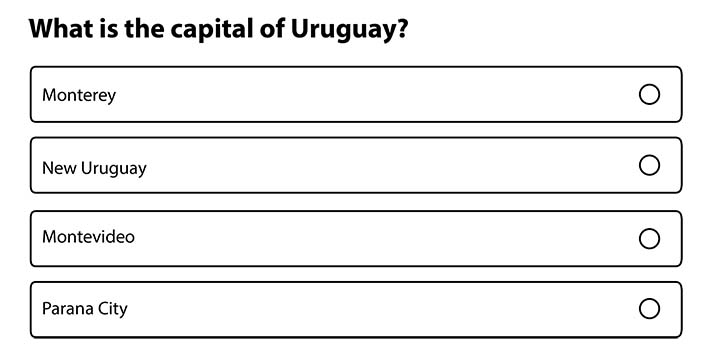This screenshot captures a potential question from an online test interface. The screen features a clean, white background with prominent black, bold text positioned at the top, presenting the question, "What is the capital of Uruguay?" Beneath the question are four answer choices, each enclosed within rectangular white boxes with black outlines. To the right of each box is a clickable circle for selection. The dimensions of these answer boxes are approximately one inch in height and six inches in width. The available answers are listed as follows: 

1. Monterey
2. New Uruguay
3. Montevideo
4. Parana City

The text for each answer resides on the left-hand side within the boxes, appearing in black and in a slightly smaller, non-bold font.